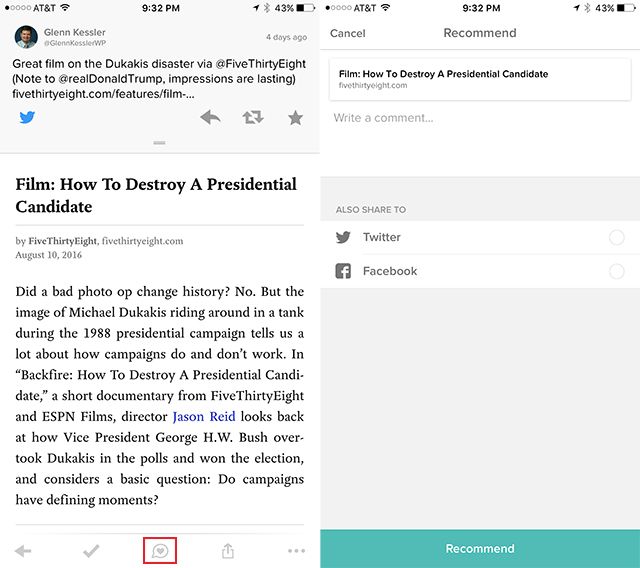The image portrays two smartphone screenshots placed side by side. 

**Left Screenshot:**
- At the top-left corner, the carrier name "AT&T" is visible.
- The time is displayed in the center as "9:05 p.m."
- On the right-hand side, the signal strength indicator and battery level (48%) are present.

**Right Screenshot:**
- The top bar mirrors the left screenshot with "AT&T," the time "9:13 p.m.," and the battery level at 48%.
- A Twitter post is centered, featuring a profile picture of Glenn Kessler. His handle, "@GlennKesslerWP," is noted along with the timestamp "four days ago."
- The tweet reads: "A great film on the Dukakis disaster via 538 [note to @realDonaldTrump: impressions are lasting]." A link to "538.com" is included.
- Below the tweet, an embedded article titled "How to Destroy a Presidential Candidate by 538.com, 10th August 2016" is displayed.
- The article description explores the impact of an infamous photo op during Michael Dukakis' 1988 presidential campaign, discussing the role of such events in campaign dynamics. It promotes the short documentary, "Backfire: How to Destroy a Presidential Candidate," directed by Jason Reed, produced by 538 and ESPN Films.
- A "Recommend" button is on the right and a "Cancel" button on the left, though the context of these buttons is unclear.
- Underneath the article, there is a text box inviting users to "Write a comment," which is currently empty.
- At the bottom of the right screenshot, a grey box provides sharing options for Twitter and Facebook, but no action has been taken.

Overall, the screenshots combine elements of social media and news article visuals, capturing a moment of digital interaction with contemporary political content.